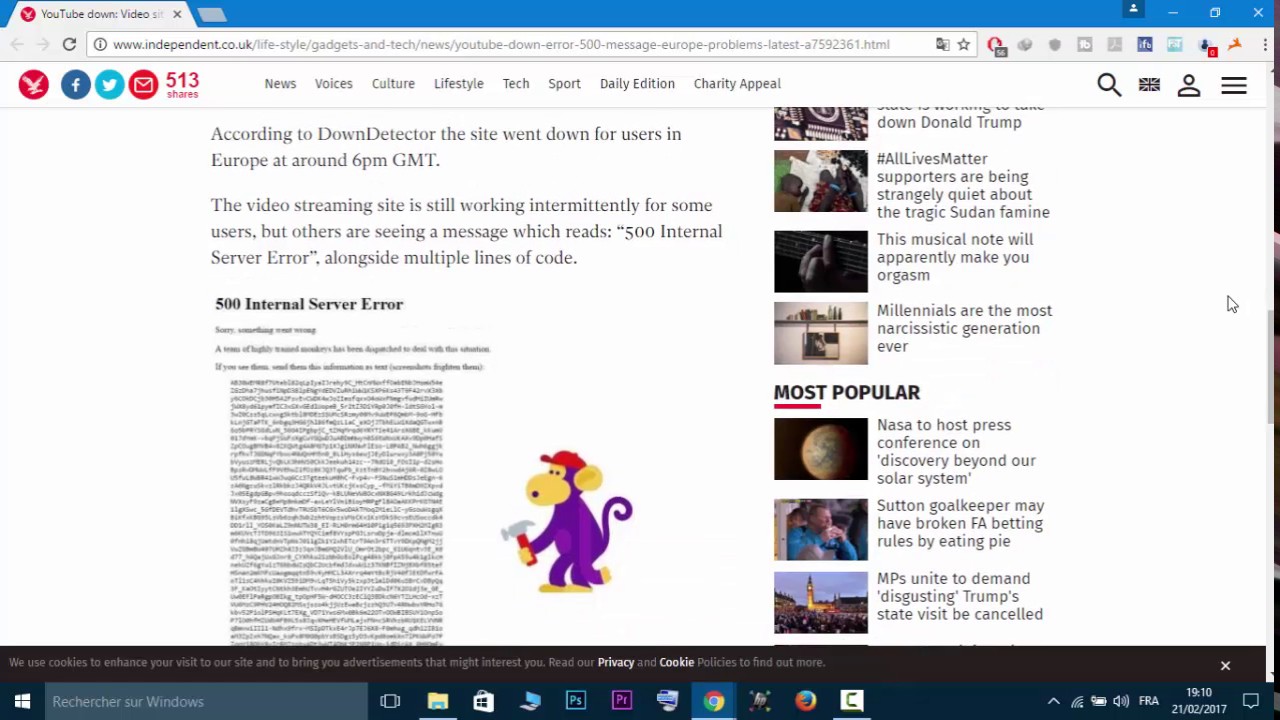**Caption:**
A detailed screenshot from the website independent.co.uk displays a 500 Internal Service Error page. The error page notably includes a whimsical illustration of an animated purple monkey holding a red hammer and wearing a red cap, positioned on the right side of the screen. The page's main text reports that, according to DownDetector, the site experienced an outage for users across Europe around 6 PM GMT. It further states that while the video streaming service is intermittently accessible for some, others are encountering an extensive list of error codes. Additionally, a column on the far right features a variety of topics covered by the site, including "All Lives Matter," discussions on millennials and cultural themes, and scientific announcements like NASA's upcoming press conference on a discovery beyond our solar system.